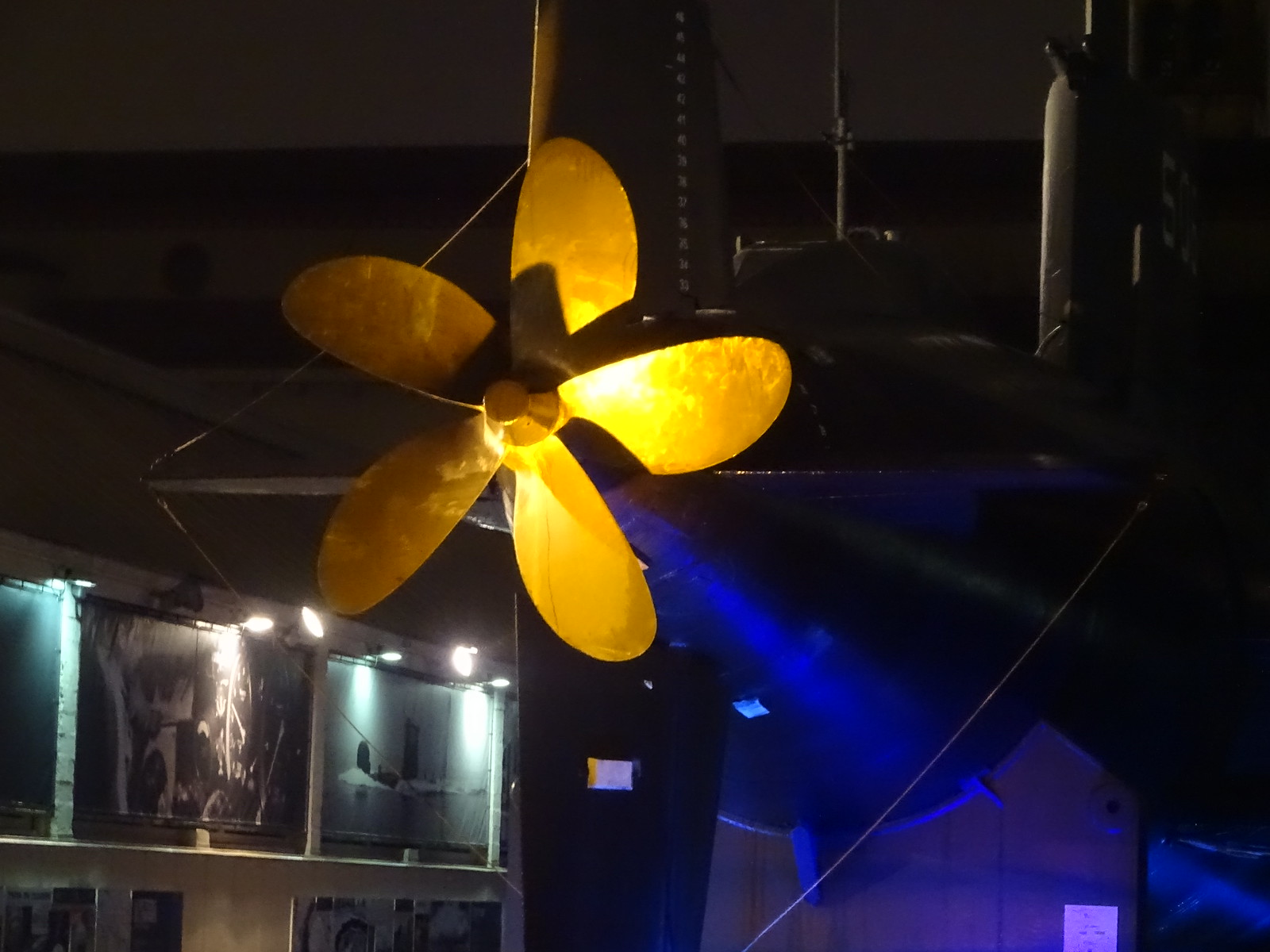This detailed indoor photograph captures a striking exhibit in a museum, showcasing a large model of a submarine. Dominating the left-center of the frame is a vivid, five-bladed golden propeller, illuminated by spotlights that cast dramatic shadows and reflections, highlighting its polished surface. The propeller is attached to the rear of the submarine model, which features an upside-down T-shape structure and a cylindrical body extending forward, tinted slightly blue by the lighting. Above this, rectangular fins and a conning tower are visible, indicating the submarine's streamlined design.

Suspended from the ceiling by guide wires, the submarine model is presented in a spacious, two-level exhibition area. The walls are a blend of brown and gray tones, adorned with black-and-white photographs and various displays related to submarines and their history. The photographs, some depicting submarines and others showing crew members, are individually lit by targeted spotlights. Metal scaffolding along the walls adds to the industrial aesthetic of the space, which is characterized by a stark contrast between the well-lit displays and the shadowed, dark ceiling. The photograph is crisp, capturing the intricate details of both the submarine model and its surrounding environment.